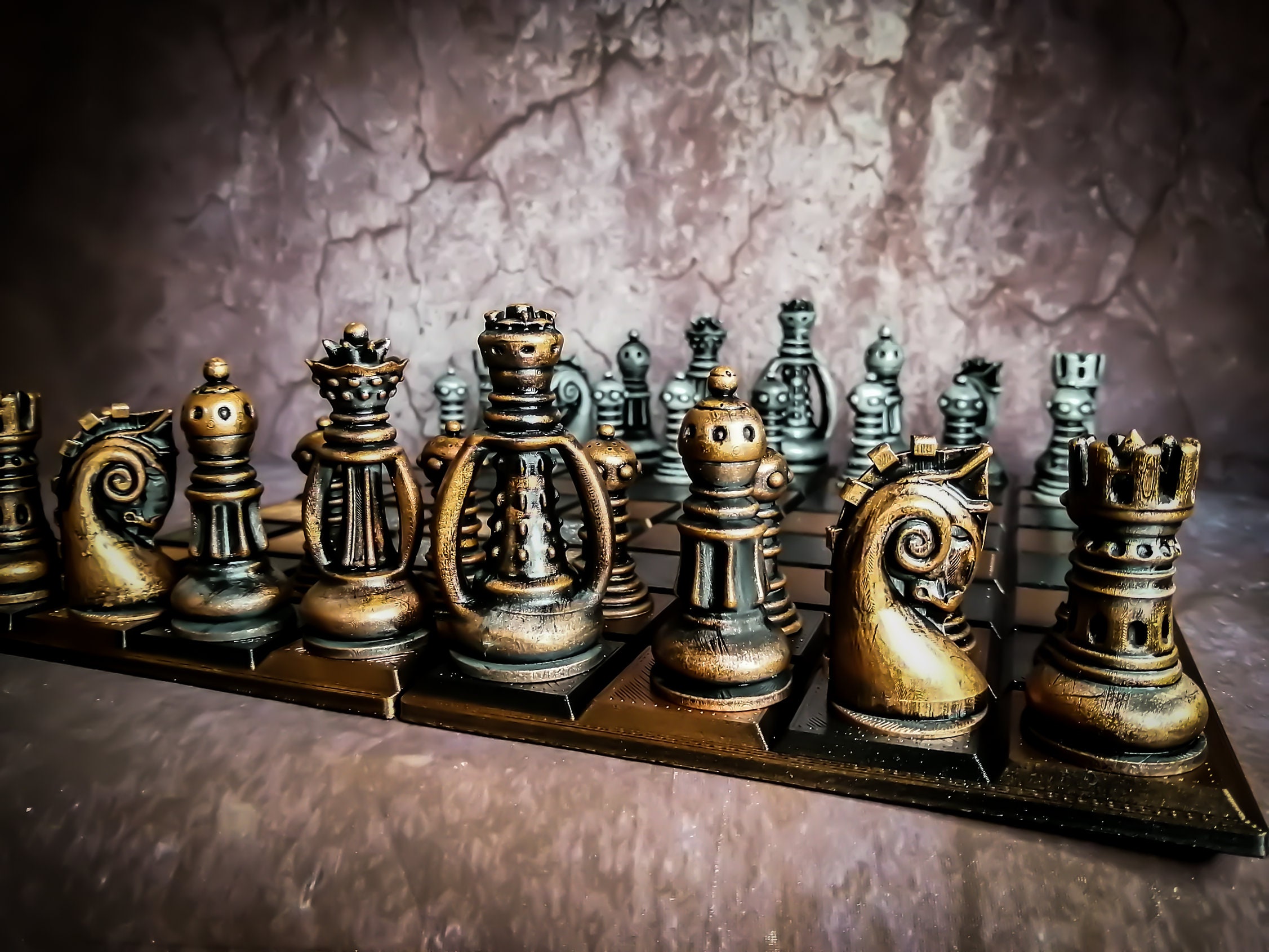This photograph captures a highly ornate and antique chess set, characterized by its two distinct sets of chess pieces. In the foreground, eight bronze-colored pieces line up, showcasing extensive detailing and a mechanical design. These pieces feature black accents and suggest their old age through visible tarnish. The chessboard, predominantly dark brown with gold and black squares, sits on a purple surface embellished with black lines. Surrounding the board is a decorative lining with white dots. In the background, the opposing set of pieces is silver with black accents, and although slightly out of focus, their intricate design is still noticeable. The blurred backdrop resembles a rock wall, with white and black markings. The photograph is taken from a close-up angle, giving prominence to the detailed craftsmanship of the bronze pieces while providing a glimpse of the silver pieces stretched out behind them, adding depth to the image.